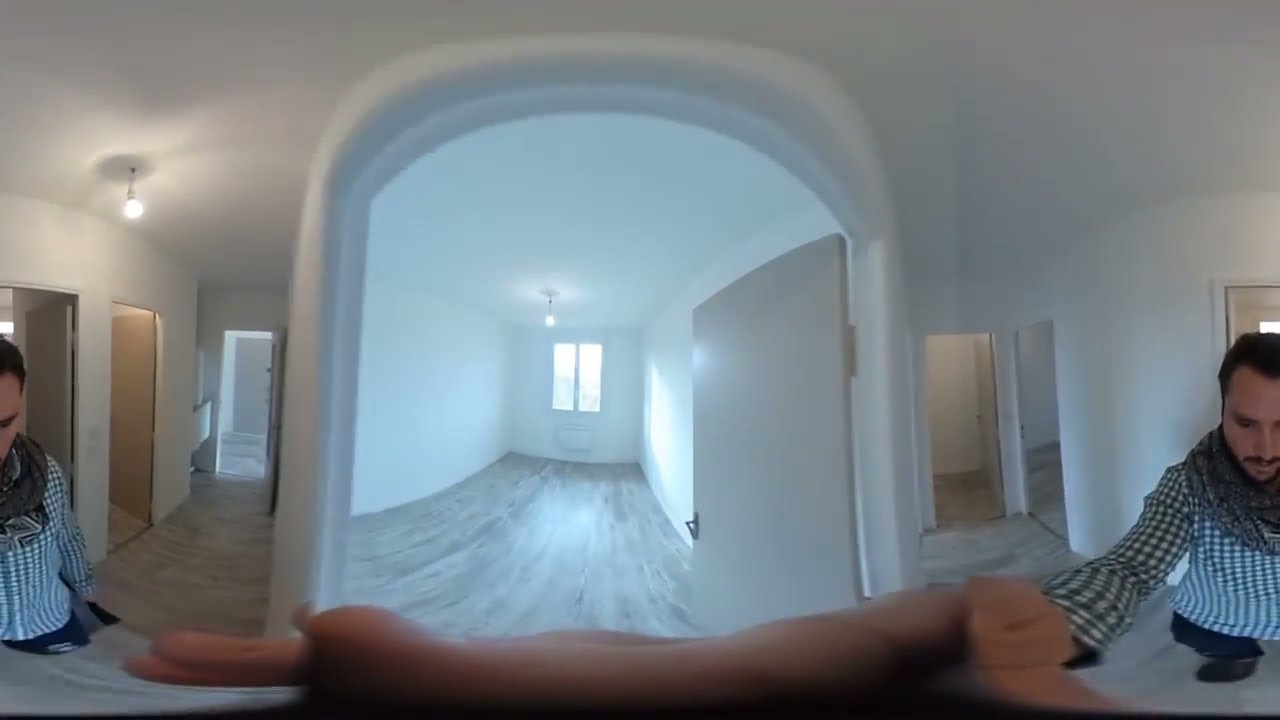The image showcases a distorted, wide-angle, possibly VR 360-degree or fisheye lens view of an unfinished apartment or house interior. Dominating both the lower left and right sides stands the same man, dressed in a blue and white checkered shirt, sporting a gray scarf, black hair, a beard, and a mustache. His hand, stretched toward the camera, becomes exaggerated due to the lens effect, covering a significant portion of the image.

The style of the photo suggests either a double exposure or a stitched panorama, making it appear as though the man is in multiple positions simultaneously within the same space. The room features white walls, a simple bulb hanging from the ceiling, and dark wooden floors. In the middle is a large archway with an open door, not mirrored symmetrically. The scene reveals multiple corridors and doorways leading to various rooms, hinting at a spacious, unfurnished interior, possibly a new construction or a home for rent. Bright sunlight streams through a window, casting light on a radiator beneath it. Despite the repetitive elements, the image provides a comprehensive, albeit surreal, view of the home’s interior layout.